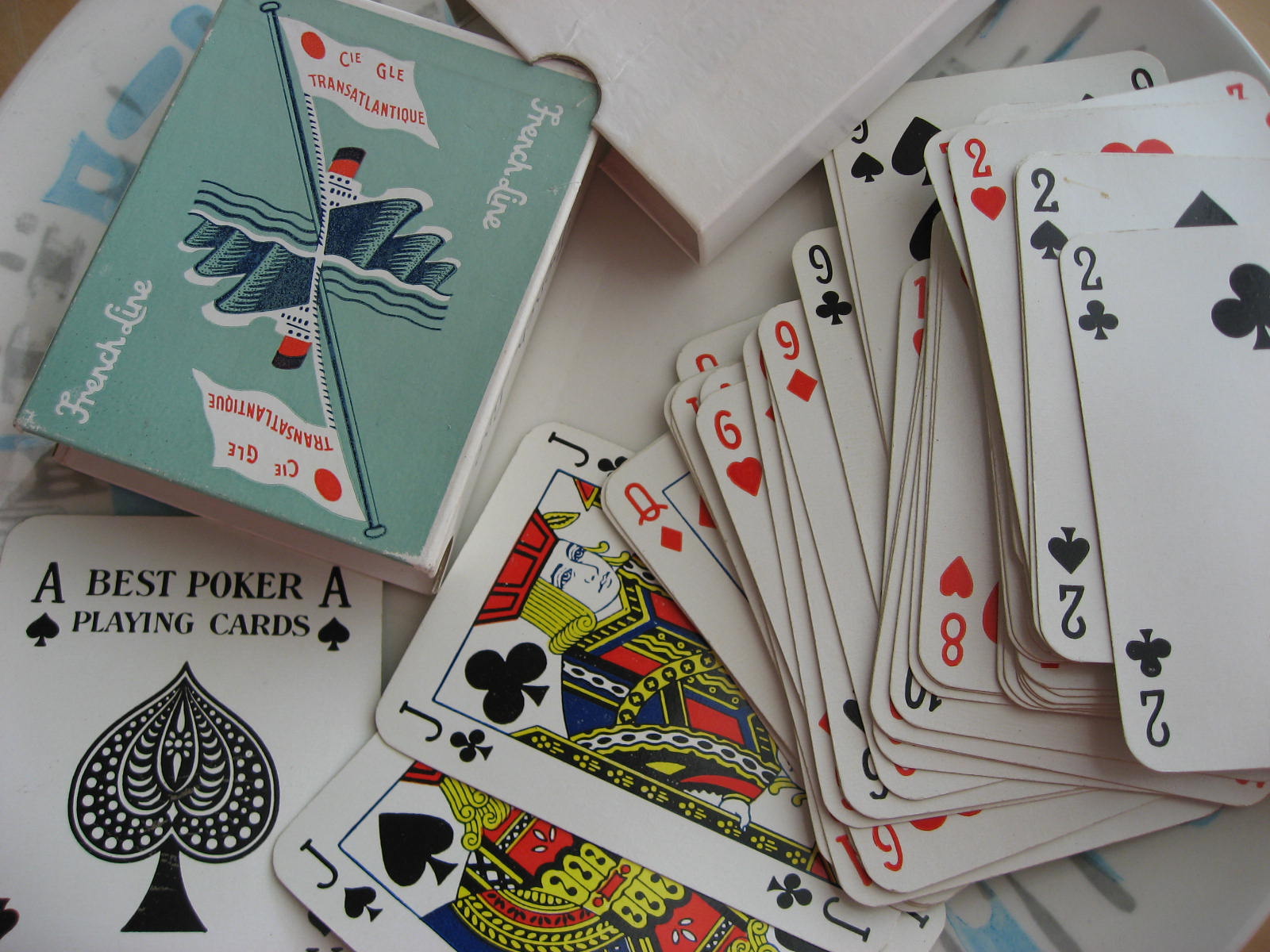In this image, a deck of cards is prominently displayed with the cards scattered over a surface. The card box is white with a semi-circle cutout at the top for easy access to the cards. The upper portion of the box is green and features the illustration of a ship adorned with a red smokestack that has a black top. The ship also bears a white flag with a red circle. On the box, the words "C-I-E-G-L-E, Transatlantic" are inscribed in orange letters, while the side of the box reads "French Line" in white letters. 

The cards are spread out on what appears to be a white tablecloth, which features distinctive blue and gray markings, including an upside-down blue exclamation point, a blue square, and some additional gray lines. Among the scattered cards, notable ones include the Ace of Spades, which is marked with "Best Poker Playing Cards" in black text. Other visible cards are a Jack of Spades, a Jack of Clubs, a Queen, a Six, three Nines, three Twos, and part of an Eight.